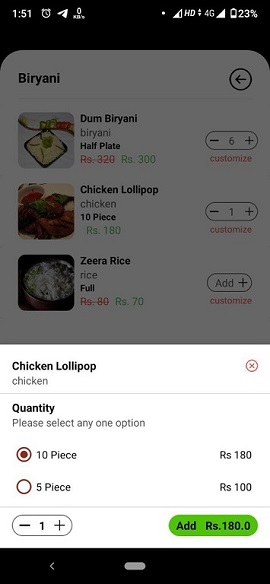The screenshot showcases a mobile phone interface, with the screen divided into two distinct sections. The upper portion has a dark gray background while the lower segment appears white. In the top right corner, the device's status indicators reveal a battery life of just 23%, full volume, and three-fourths Wi-Fi connectivity, accompanied by an "HD" label. The main content of the screen suggests the user is browsing a restaurant site, specifically looking at a menu for "Biryani." The screen displays three different chicken dishes, prominently highlighting one labeled "Chicken Lollipop." The user has selected the 10-piece portion of this dish, denoted by the quantity set to one. The price for this selection is displayed as RS180.0, likely in the local currency. Below this, a lime green "Add" button is visible, inviting the user to confirm their selection. A red action bar is located further down, presumably for finalizing the order or adding items to a cart.